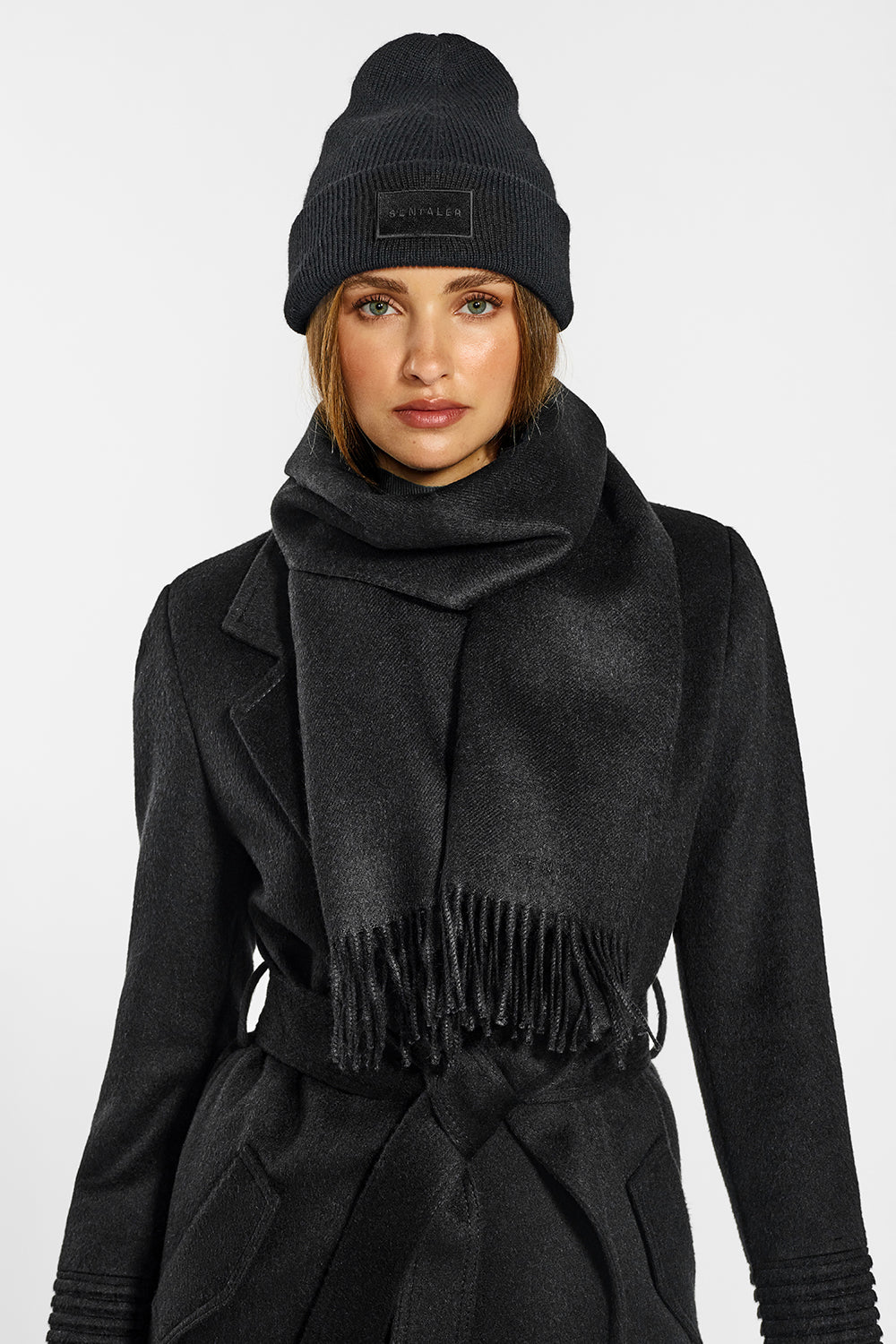The image depicts a stylish female model of Caucasian descent, photographed indoors against a light gray background. She appears to be showcasing winter wear, including an all-black ensemble. The model has light brown, almost shoulder-length hair framing her face, and she is wearing makeup with greenish-blue eyes and red lipstick. She dons a black stocking hat labeled "Centaler" just above her eyebrows, and a matching black scarf with tassels that drapes down to her waist. Her outfit features a long-sleeved, solid black coat with a wide lapel and a twist-tied belt at the waist, which has pockets on the lower half. The image is cropped to show her from about the hips up, with the background providing a clean contrast to her dark attire.